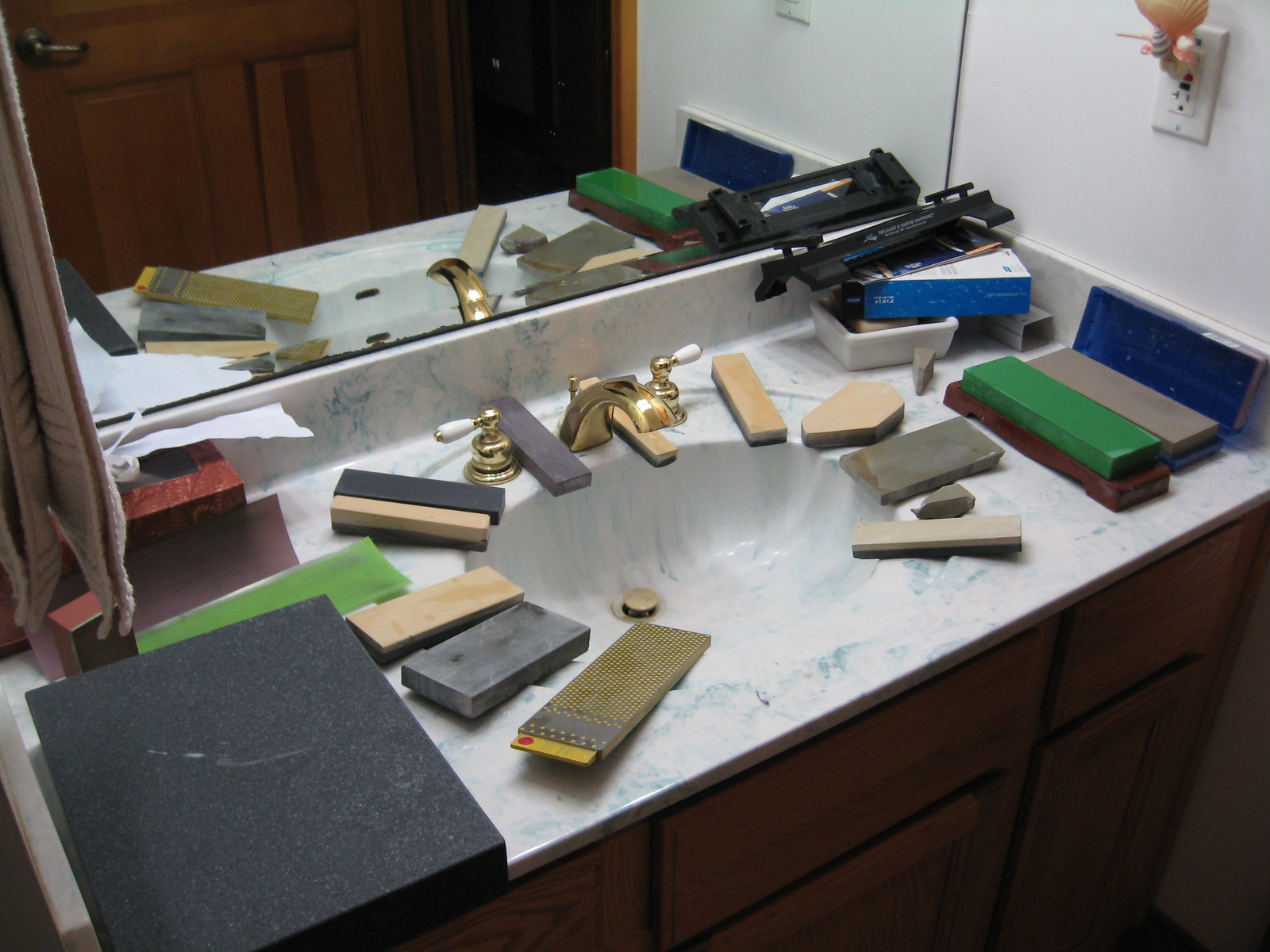The image captures a detailed view of a sink countertop vanity. Centered at the top is a large mirror, reflecting the elements on the sink below. To the right, a brown wooden door with a horizontal handle is visible. The walls around the vanity are painted white. In the upper right corner of the image, there are two electrical outlets, each equipped with black and red reset buttons.

A pink snail-shaped nightlight is affixed to one of the outlets. The sink itself is made of white marble with blue streaks and features a sunken basin that blends seamlessly with the countertop. The faucet is made of gold, with handles that are gold with white tips. 

Currently, the sink is turned off. The countertop is cluttered with various rectangular blocks, either made of wood or stone, arranged in a semi-circular pattern around the sink. Additional blocks are scattered on the sink, suggesting that the user might be working on a project involving these materials or is in the process of cleaning them.